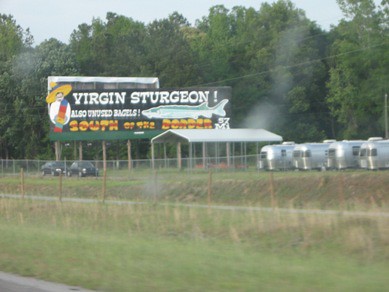In the foreground, a serene field stretches out, bordered by a quaint road running parallel to it. A wooden fence demarcates the field, and beyond it, another road is visible. To the side of the field, a series of airline trailers are parked under a shelter, providing a subtle, industrial contrast to the pastoral scene. Dominating the background, a large black billboard catches the eye. The lower portion of the billboard is green, and the top part features bold white text that reads "Virgin Sturgeon!" Below, it advertises "unused bagels." The right side of the billboard is adorned with an image of a sturgeon fish, while the left side features a man wearing a sombrero and a colorful, rainbow-striped cape draped over his shoulder. Beneath this character, vibrant yellow text with a red slash across it declares "South of the Border." Framing the entire scene, lush trees rise up in the distance, adding a touch of natural beauty to the eclectic mix of elements in this vivid tableau.